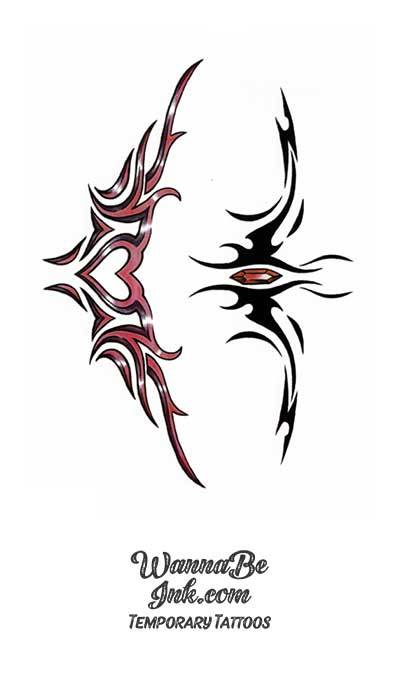The image features a heart-shaped design at its center, flanked by two vertical elements set against a white background. The left side of the image is primarily pink, showcasing a sideways heart with floral or leaf-like, ribbon-shaped elements emanating from it, resembling flames. On the right side, there is an abstract black shape with curved lines, featuring a faceted, gemstone-like hexagon in its center. Below these artistic elements, the text "WannabeInc.com Temporary Tattoos" is written in black cursive font, emphasizing the temporary tattoo business logo style.